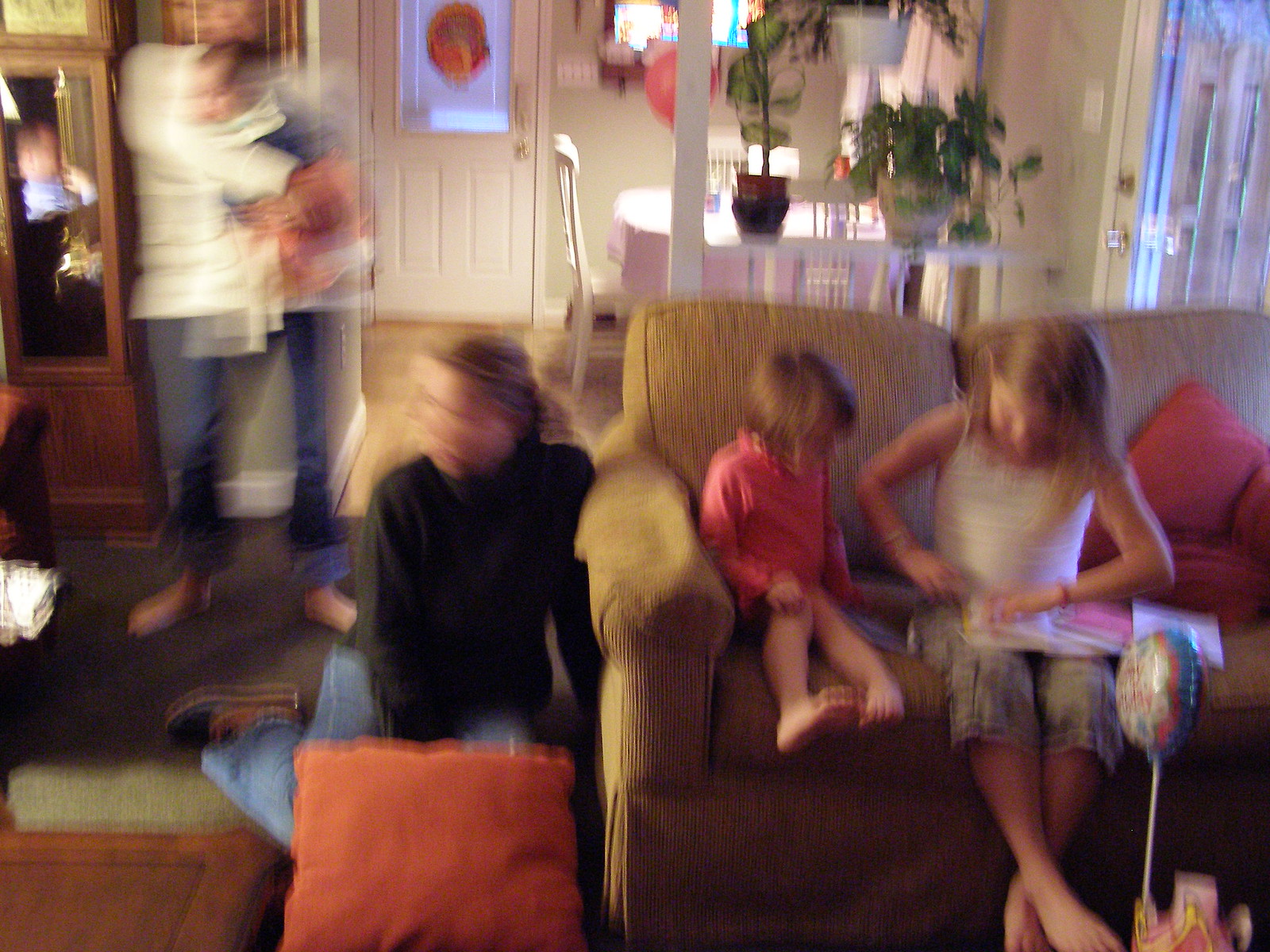In this image of a family gathering, albeit extremely blurry, we can see an 80s-style home interior. Central to the scene is a brown couch where two young girls are seated. The elder, appearing around seven to eleven years old and dressed in calf-length pants and a white T-shirt, seems to be opening a gift or looking through a photo album, while the younger toddler, in a long-sleeve red shirt, watches intently. To the right of the couch, a blonde-haired woman—likely their mother—is kneeling on the hardwood floor beside an orange pillow, her face turned slightly away but appearing to smile. In the backdrop, an older woman in blue pants and a white shirt stands near a kitchen table accompanied by potted ivy plants. A grandfather clock leans against the wall in the background, and to the right, a stick balloon is visible at the bottom corner. The living room exhibits a mix of hardwood and tiled flooring, with a grey rug near the front door. A man and possibly another woman holding a baby are vaguely present in the background amidst the house's elements, which include throw pillows in brown, rust, and reddish tones.